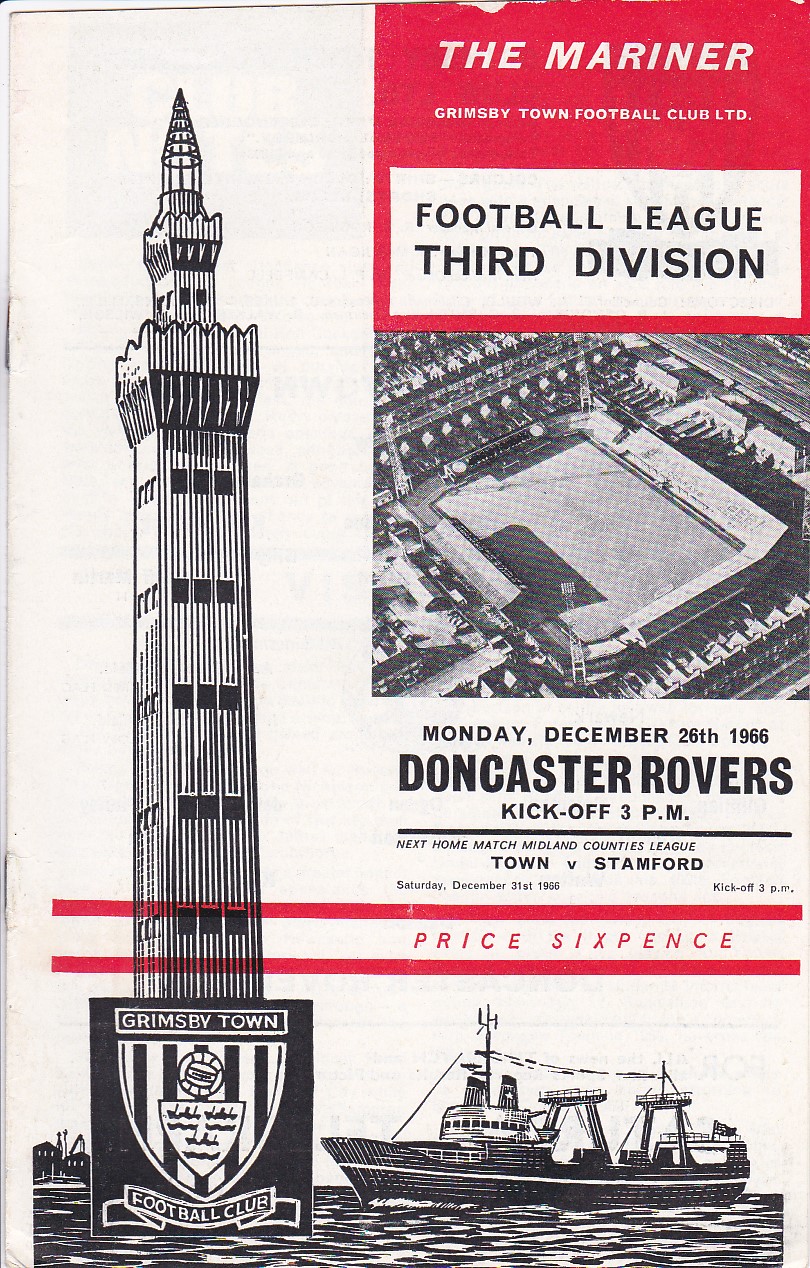The image is an aged, worn cover of an old sports program for the Grimsby Town Football Club in the Football League, 3rd Division. The cover, designed in black-and-white pen illustration, features a tall, skinny structure that appears to be a lighthouse, with a body of water and a ship at the bottom. Between the lighthouse and the ship is the Grimsby Town Football Club’s logo, which includes a shield with a soccer ball in it. The top portion of the cover prominently displays the title "The Mariner." Details of an upcoming game against the Doncaster Rovers are written in a red box with white letters, specifying the date as Monday, December 26, 1966, with a kickoff at 3 p.m. The price of the program is listed as sixpence. Additionally, there is a black-and-white photo of the stadium where the match will take place.